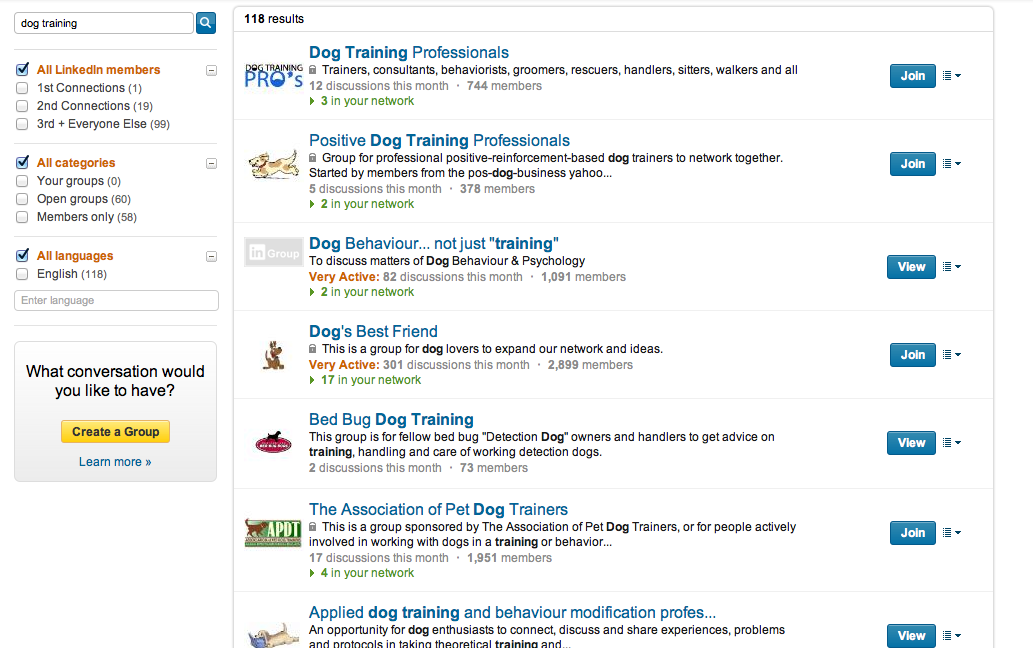On the left-hand side of the image, there are two rectangles. The first rectangle contains a search bar that is predominantly white with black text. The search bar has the text "dog training" written in it. Adjacent to the search bar, there's a blue square featuring a white magnifying glass icon. Below these elements, a thin gray line runs horizontally across the rectangle.

Beneath the gray line, the text is formatted in various colors and sections:

- In orange, it states "All Linked Members" with a checkbox next to it.
- In black, it lists the connection types: "First Connections," "Second Connections," "Third," and "Everyone Else."
- In orange, it says "All Categories."
- In black, there are additional options: "Your Groups," "Open Groups," "Members Only."
- It mentions "All Languages" in or to Armish, accompanied by a checkbox.
- The language selection further specifies "English."

The second rectangle is mostly gray with sections of black text. It prompts, "What conversation would you like to have?" Below this prompt, there's a yellow section with black text that reads "Create a Group." Underneath that, there's a blue section with the text "Learn More."

The main portion of the image is dominated by a large white search box with the text "118 results" written in black. Following this, a series of group names and descriptions are listed:

- A blue section with the text "Dog Training Professionals." Underneath this, it lists various roles in black text: "Trainers, Consultants, Behaviorists, Groomers, Rescuers, Handlers, Site Workers, and All." Next to this section, there's a blue box with white text that says "Join."
- Another entry in blue text reads "Positive Dog Training Professionals," with an adjacent blue box having white text that says "Join."
- Following this, additional group names are listed in blue: "Behavioral, Not Just Training," "Dog Best Friends," "Bed Bug Dog Buddies Training," "The Association of Pet Dog Trainers," and "Apply Dog Trainer Behavior Modification Professionals."

The last three entries each feature a blue box with white text that says "View."

The overall image appears to be a user interface for searching and joining various dog training professional groups, categorized clearly and with options for membership and interaction.